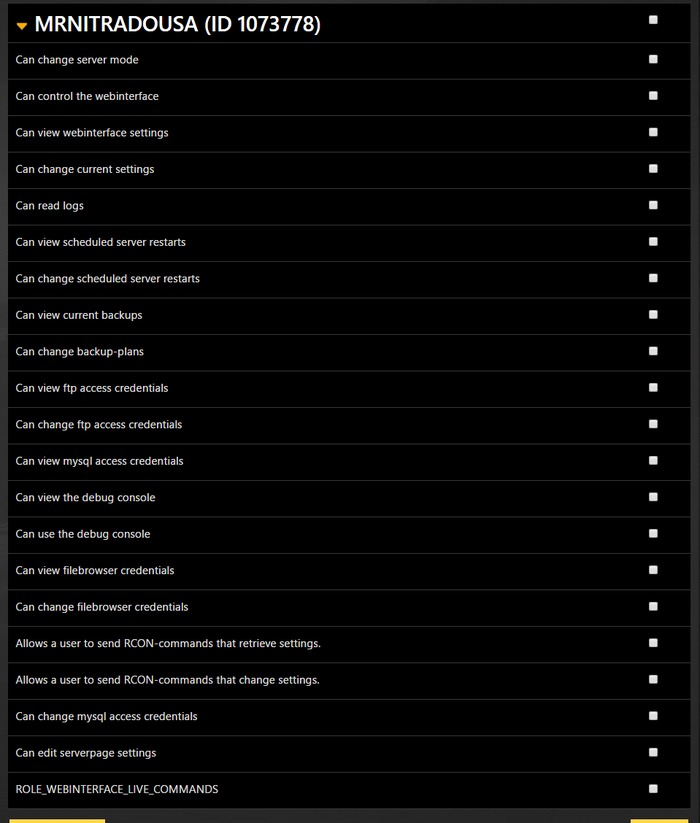The image depicts a detailed administrative configuration page, featuring a series of text descriptions and corresponding checkboxes, presented in white text against a black background. At the very top, the page is titled "Marintra Doza" with the identifier "ID 1073-778" in parentheses. Each line item on the page includes a specific permission description followed by an empty white checkbox, allowing for selection.

The permissions listed are as follows:
1. Can Change Server Mode
2. Can Control the Web Interface
3. Can View Web Interface Settings
4. Can Change Current Settings
5. Can Read Logs
6. Can View Scheduled Server Restarts
7. Can Change Scheduled Server Restarts
8. Can View Current Backups
9. Can Change Backup Plans
10. Can View FTP Access Credentials
11. Can Change FTP Access Credentials
12. Can View MySQL Access Credentials
13. Can View the Debug Console
14. Can View File Browser Credentials
15. Can Change File Browser Credentials
16. Allow a User to Send Archon Commands that Retrieve Settings
17. Allow a User to Send Archon Commands that Change Settings
18. Can Change MySQL Access Credentials
19. Can Edit Server Page Settings
20. Roll_Web_Interface_Live_Commands

The bottom of the page features several yellow bars. These elements likely represent additional interface components or status indicators, though their exact purpose isn't clearly defined in the image description.